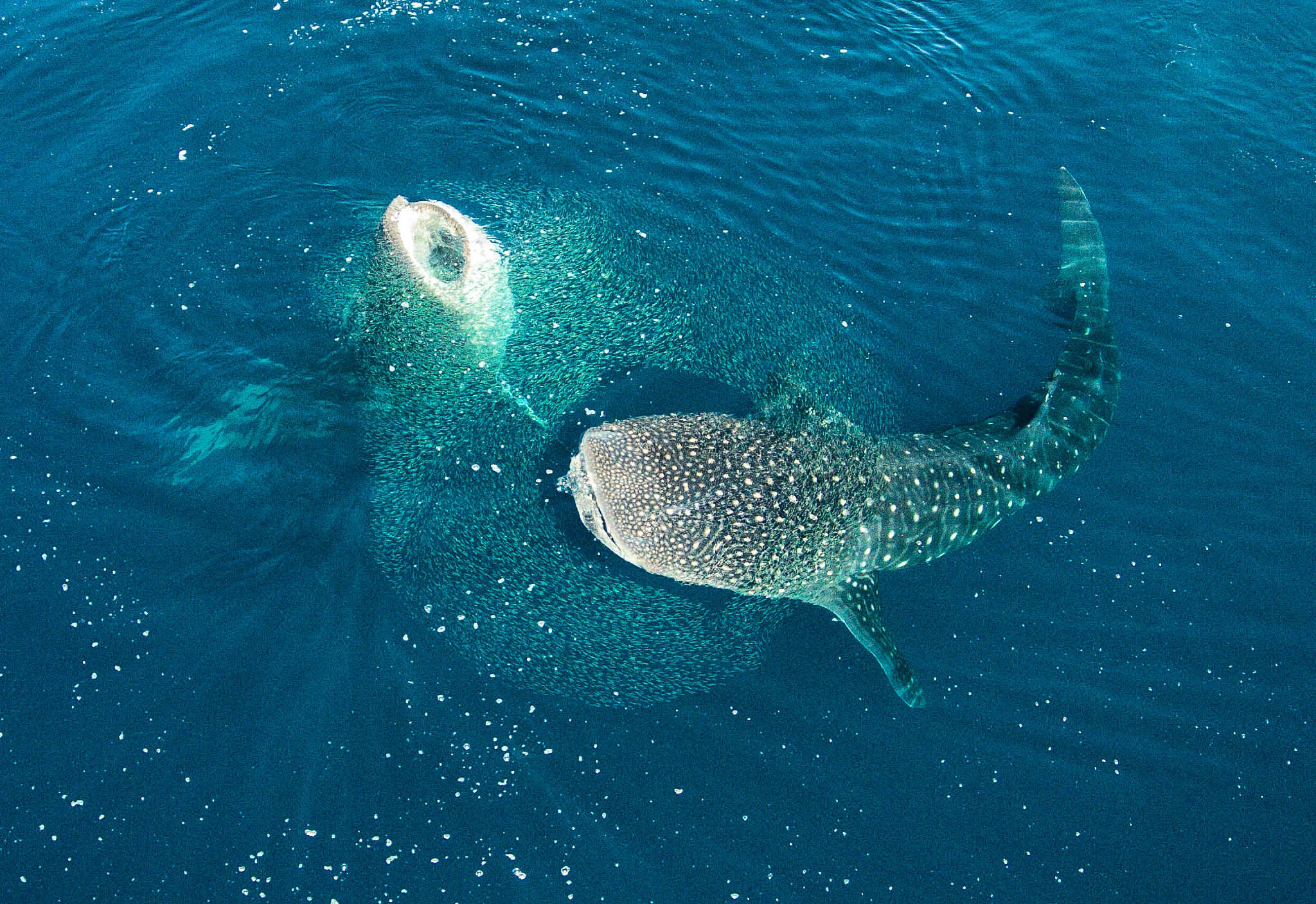This overhead photograph captures a stunning view of the deep blue ocean, punctuated by flecks of white foam. At the center of this vibrant scene are two large sea creatures, distinguishable by their markings and posture. On the left, a whale emerges with its broad, rounded nose pointed upwards and its dark gray body covered in densely packed white speckles. Its curved tail arcs gracefully, creating a dynamic, slightly curved shape. To the right, a shark is captured mid-leap, its open mouth revealing a glimpse of its white belly. The shark's body is adorned with a unique polka dot pattern, denser towards the head and more sparse towards the tail. The water around them is alive with movement, rippling and swirling as evidence of their interaction. The overall composition emphasizes the contrast between the serene blue of the ocean and the dynamic presence of these majestic marine animals.